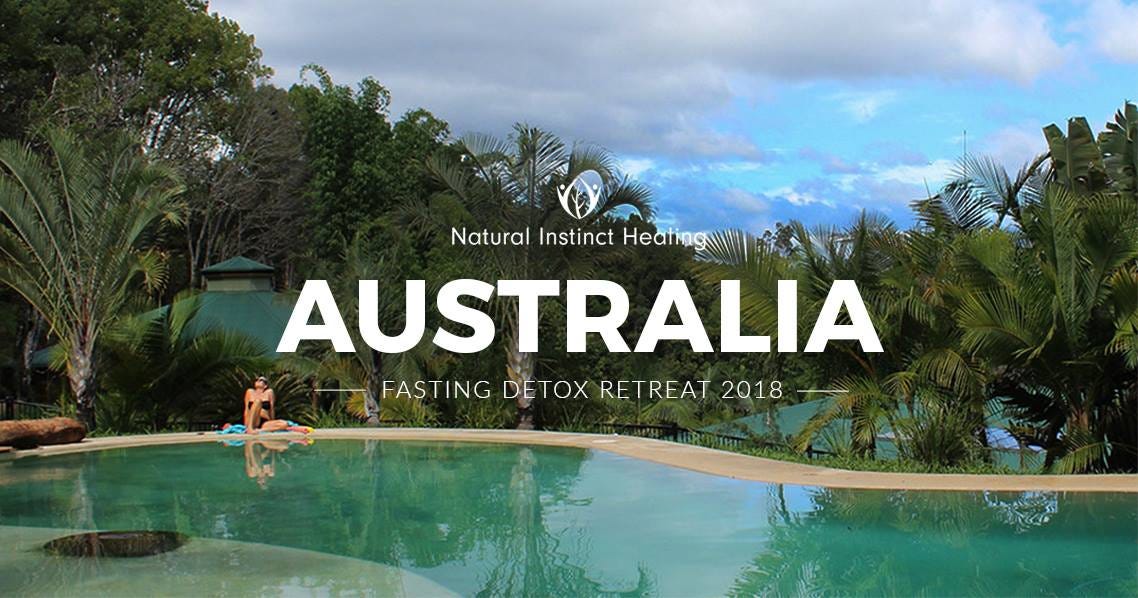This image is a rectangular photograph turned into an advertisement, measuring about five inches wide and three inches high. It features an outdoor daytime scene at a tropical resort. A kidney-shaped swimming pool with blue-green water, reflecting the surrounding greenery, dominates the lower third of the image. The pool’s light brown deck curves in an S-shape, wrapping around from the bottom corners and meeting in the center.

A woman sits on the left side of the pool, sunbathing on a blue towel. She is wearing a black bikini and is leaning back on her hand. Behind her, lush green palm trees rise up, and the green roofs of buildings are partially visible through the foliage. In the upper right corner, a light blue sky with grayish-white clouds stretches across the background. 

Overlaying the center of the photograph, white text promotes an event. It reads, "Natural Instinct Healing" followed by "Australia" in larger bold letters and "Fasting Detox Retreat 2018" in smaller print below. The thoughtful placement of text and the serene tropical setting create an inviting atmosphere for the advertised retreat.